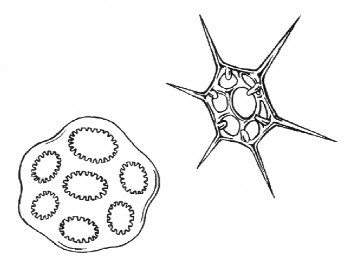This black and white ink drawing features two distinct figures against a white background. On the bottom left-hand side, there is a large, rounded object resembling a blob. This figure has a textured surface with seven jagged, oval shapes embedded within it, each with rough edges, almost giving the impression of squiggly spikes. Lines extend from this figure to its outline, creating an intricate and organic feel. On the top right-hand side, a hexagonal shape with six sharp, elongated spikes protruding from each corner catches the eye. This star-like figure has a central circle surrounded by six ovals arranged symmetrically; additional rounded shapes or protrusions can be seen within its form, adding to the complexity. The contrast between the rounded, blobby shape and the sharp, spiky hexagon highlights the intricate detailing of these figures, resembling abstract representations of microbes or microscopic entities.